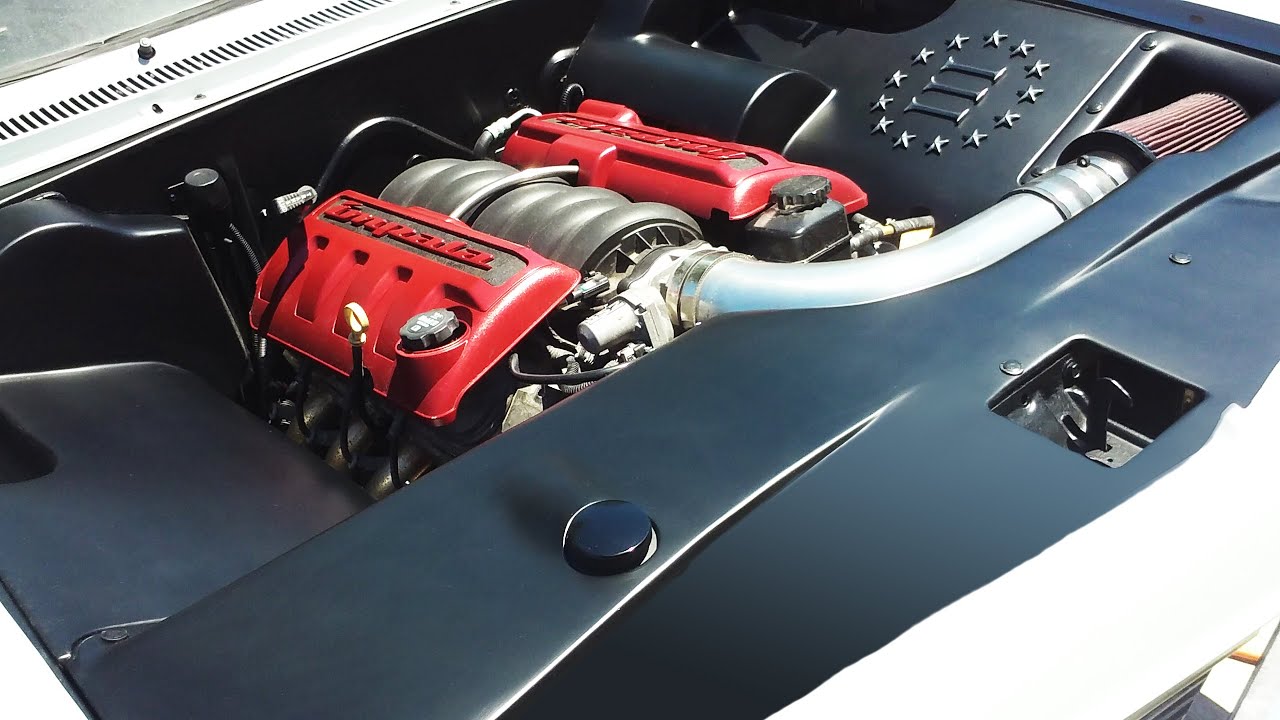The photograph captures a high-performance engine, likely a V6 or V8, with the car’s hood raised for full visibility. The engine, characterized by its striking red valve covers and silver components, appears to be exceptionally clean and features distinct high-performance elements. Notably, it includes a supercharger atop the manifold, with an air filter attached to one of the fender wells. Prominently displayed on one of the side panels is a symbol—a Roman numeral three encircled by stars—whose significance is unclear. The image suggests meticulous details such as an area to check the oil, a probable transmission fluid port, and a black push button which seems to control the engine compartment latch. The word "Impala" is inscribed in red text within a grey indented line on the engine. The photo is taken from the front left perspective of the car, allowing a slight view of the windshield at the upper left corner of the frame.